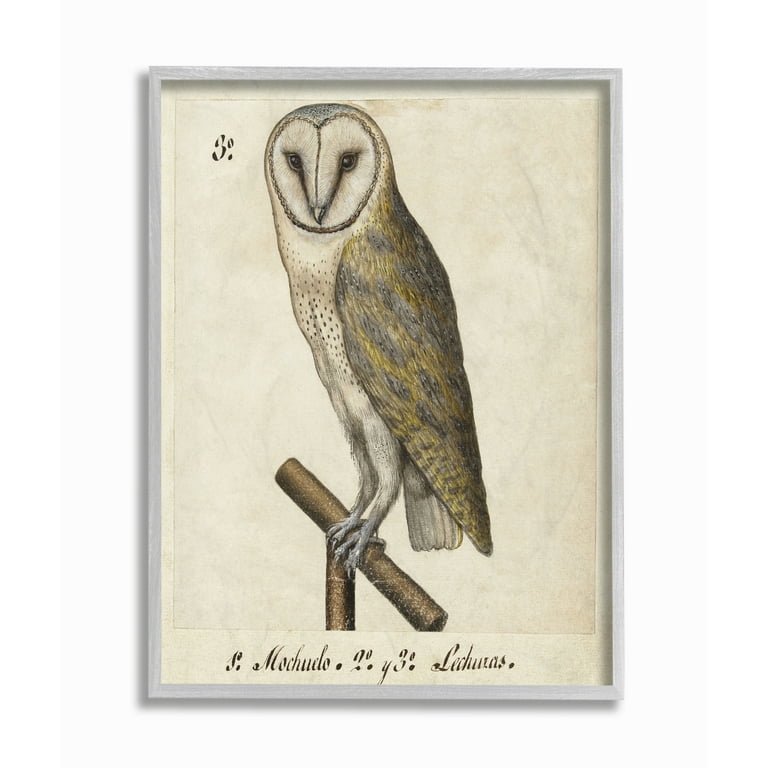The image is a detailed illustration of an owl, either crafted with pencil or ink, displayed prominently on a plain white wall. The artwork is enclosed in a simple gray wooden frame. The illustration, on what appears to be yellowed paper, features a barred owl perched on a T-shaped brown stand. The owl is rendered with a white face and body that has black spots. Its wings are a striking golden-yellow with dark brown or black textured accents. The owl’s sharp talons and big black eyes give it a piercing look directly at the viewer. Below the owl, written in script, is likely the artist's name, which reads "Mochudo Lechurus," along with some other partially legible text and numerical details in the upper left corner.